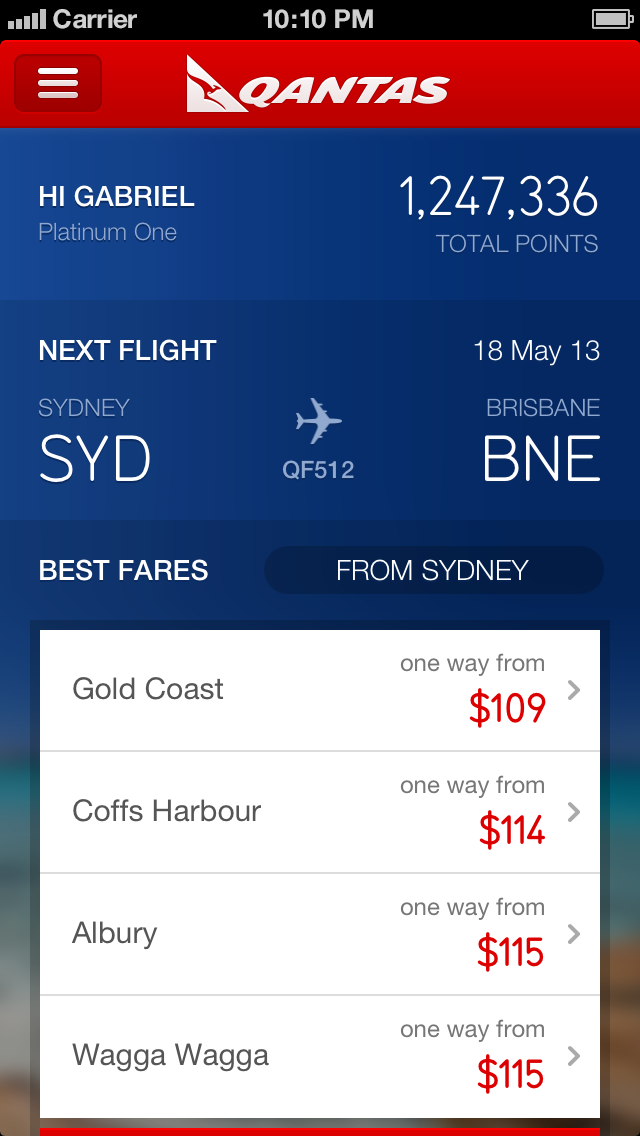On a blue background, the image features the Qantas logo in white set against a red header. At the top right corner, the time is displayed as 10:10 p.m. The screen welcomes High Gabriel, a Platinum One member with an impressive total of 1,247,336 points.

The next-flight information shows the details for flight QF 512 departing from Sydney (SYD) to Brisbane (BNE) on 18 May at 13:00.

Highlighted offers include:
- Gold Coast: One-way fares starting from $109, displayed prominently in red text within a blue-oval backdrop.
- Coffs Harbour: One-way fares starting from $114.
- Albury: One-way fares starting from $115.
- Wagga Wagga: One-way fares starting from $115.